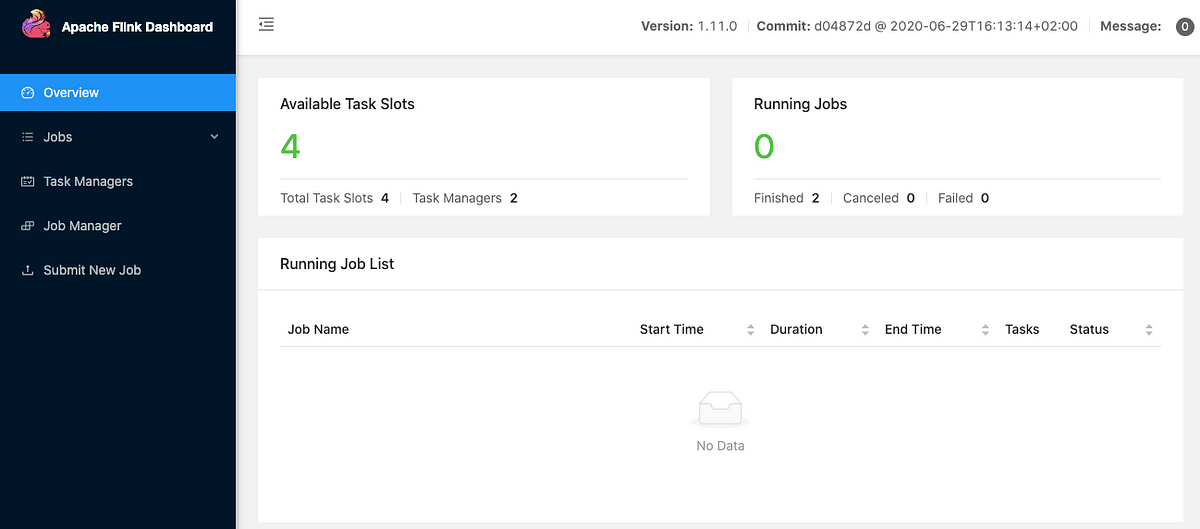The image depicts a detailed view of a webpage titled "Alpha Flank Dashboard." On the left-hand side, there's a vertical black column with a cartoon image. The black column features navigation options in blue and white, including "Overview," "Jobs," "Task Managers," "Job Manager," and "Submit New Job."

The main section of the webpage showcases the version details, stating "Version 1.1.1.0 Comet" followed by a lengthy serial number. Below this, there's a status section reporting "Messages" with a count of zero inside a gray circle. The "Available Task Slots" are prominently displayed as four in green, and similarly, "Total Task Slots" are listed as four. "Task Managers" number two.

A few performance metrics are highlighted, with "Running Jobs" at zero, and lime-green statistics indicating "Finished: 2," "Canceled: 0," and "Failed: 0."

Further down the page, a white box titled "Running Job List" provides column headers for "Job Name," "Start Time," "Duration," "End Time," and "Task Status," accompanied by up and down arrows, but no data is currently displayed. An illustration of an open envelope, which appears empty, symbolizes the absence of ongoing jobs or tasks.